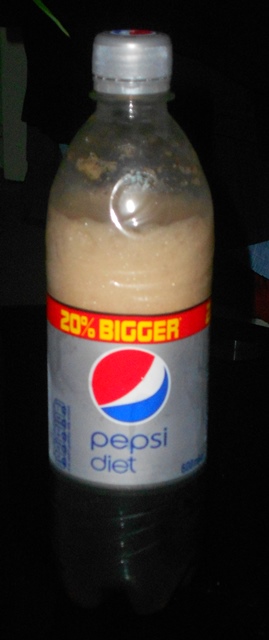The photograph depicts an individual-sized serving bottle of Diet Pepsi. The bottle, made of clear plastic, prominently features a label indicating it is 20% bigger than standard sizes, which suggests a volume above the typical 20 ounces. The base of the bottle is shadowed, creating ambiguity about its color—it could be black or just darker due to the background. The label itself is a sleek gradient of gray to silver, with the iconic red, white, and blue Pepsi logo centered. Below the logo, the text reads "Diet Pepsi." The bottle is topped with a silver cap. The contents of the bottle are not full; a significant amount of the Diet Pepsi has been consumed. The remaining soda has been agitated, resulting in a light brown foam occupying the space above the label, contrasting with the usual dark hue of the liquid.